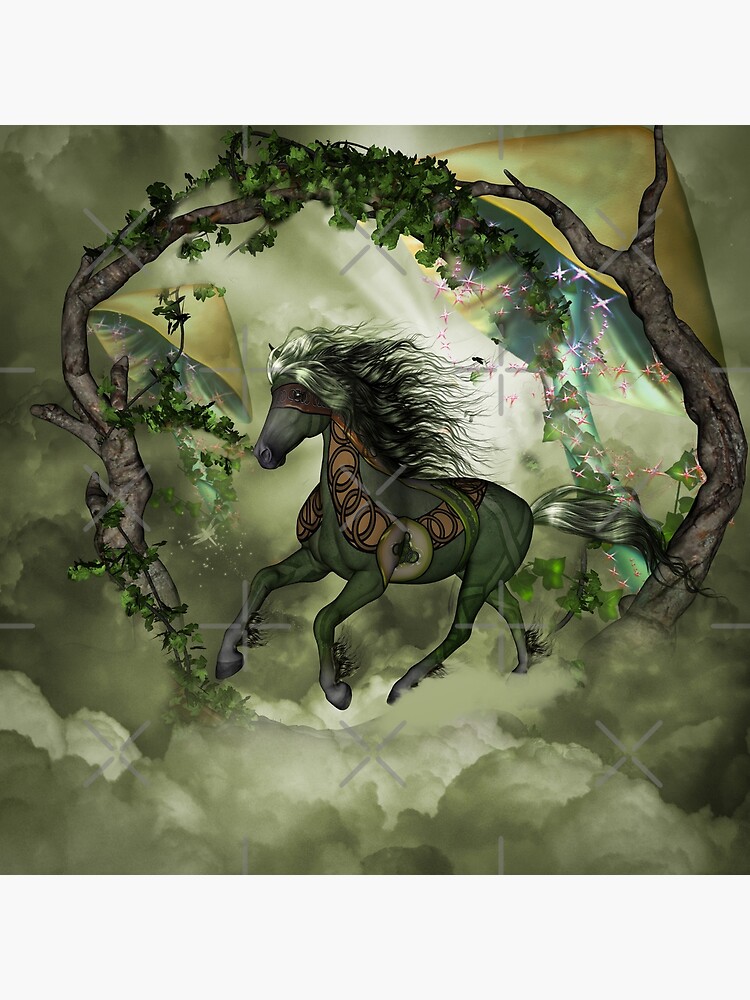This is a square, digitally illustrated image featuring an ethereal, dark green horse with a flowing mane and tail that blend shades of black, silver, and dark green. The horse, adorned with intricate interlooping rings and a brown mask over its eyes, races through verdant, puffy clouds. Encircling the horse is an archway made of intertwined branches and leafy vines, giving the impression it's moving through a natural hoop. Surrounding this whimsical scene are large, fantastical mushrooms, with two towering on the left and one on the right. A multitude of small, bright star-like elements, which could be stars, fireflies, or even dragonflies, add a magical feel. The background melds into a dreamy sky both above and below the horse, further enhancing the picture's otherworldly atmosphere. Additionally, subtle gray X's and check marks can be seen scattered throughout the image, contributing to its outlandish, fantasy-like quality.